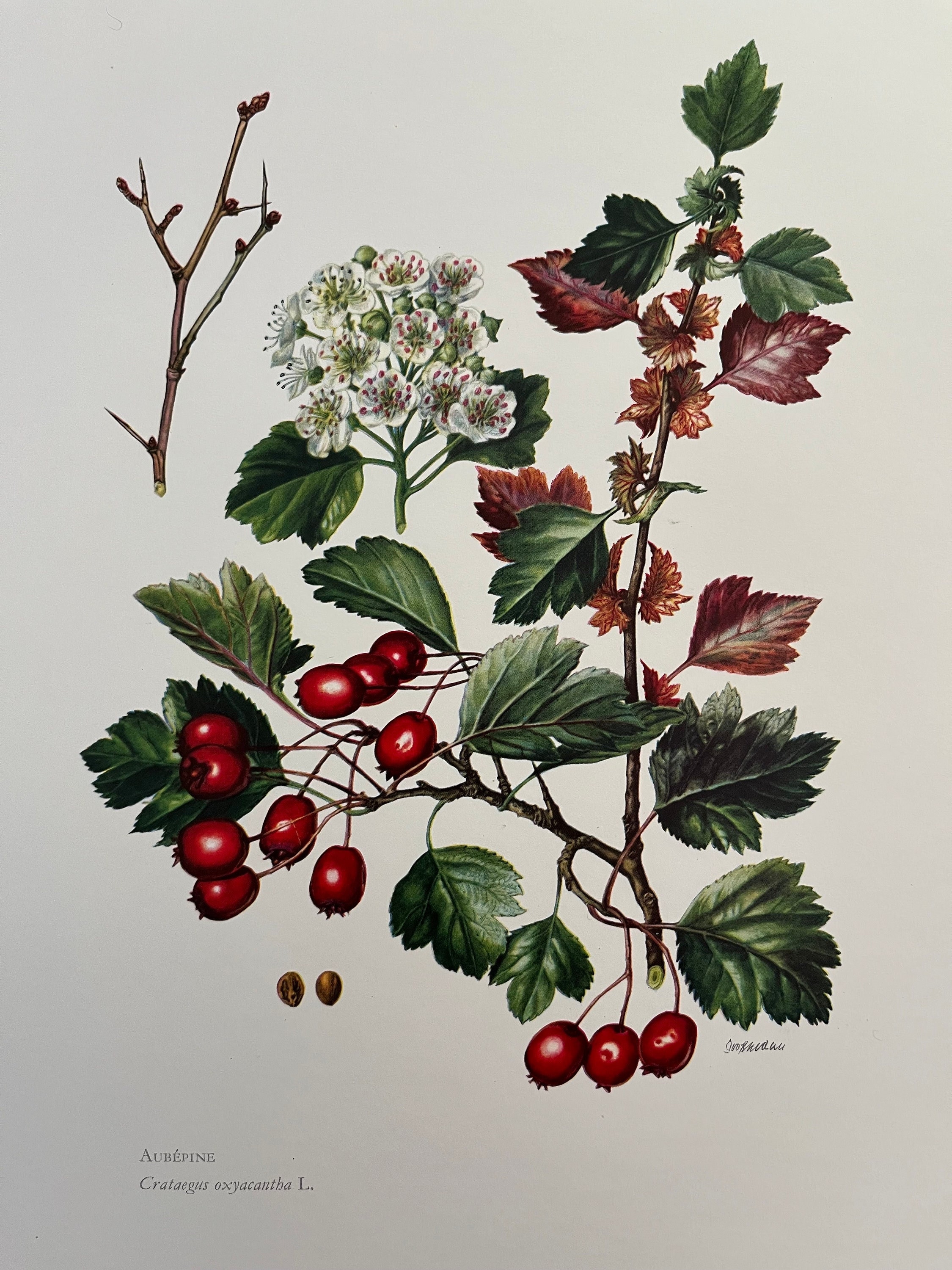This image is a strikingly detailed and realistic hand-drawn artwork of a hawthorn plant, known scientifically as Crataegus Oxyacantha, as indicated by the text "ABEB PINE CRETAGUS OXYCANTHOLE" at the bottom left. The central focus is on a prominent stem that extends upward, adorned with an abundance of leaves in varied hues including dark green, light green, red, and light orange. Clusters of spherical, red berries are scattered throughout the branches. Additionally, there are smaller, green stems featuring white flowers that are delicately speckled with red. To the left, a bare twig displays small buds where future leaves might emerge, and another brown, shiny branch without leaves emphasizes the intricate and realistic detail of the artwork.